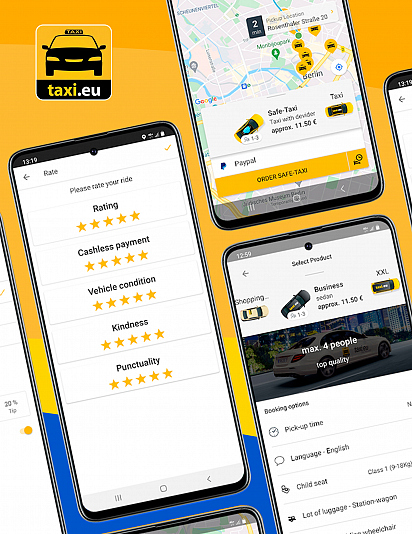This is a vertically oriented digital ad likely to appear on a website, featuring a predominantly yellow background with varying shades of yellow and a touch of white in the bottom left corner. The ad showcases three smartphones, all angled to the left, each displaying different features of a ride-share service.

In the bottom left corner of the ad, a square logo reads "taxi.eu" and displays a simplistic, black drawing of a car with a yellow detail. The phone on the far left shows a white screen with a prompt to "Please rate your ride.” It highlights several 5-star rating parameters such as rating, cashless payment, vehicle condition, kindness, and punctuality. The black phone menu bar is visible at the top of the screen.

To the right of this phone, another device is partially shown, featuring a map adorned with numerous cab icons. The screen includes the text “Safe Taxi. Order Safe Taxi” along with payment options. The third phone at the bottom displays an image of a white car and the text "Max 4 people."

A fourth phone is barely visible, cut off at the far right edge. The overall design is simple and visually pleasing, with symmetrical elements enhancing the aesthetic appeal.